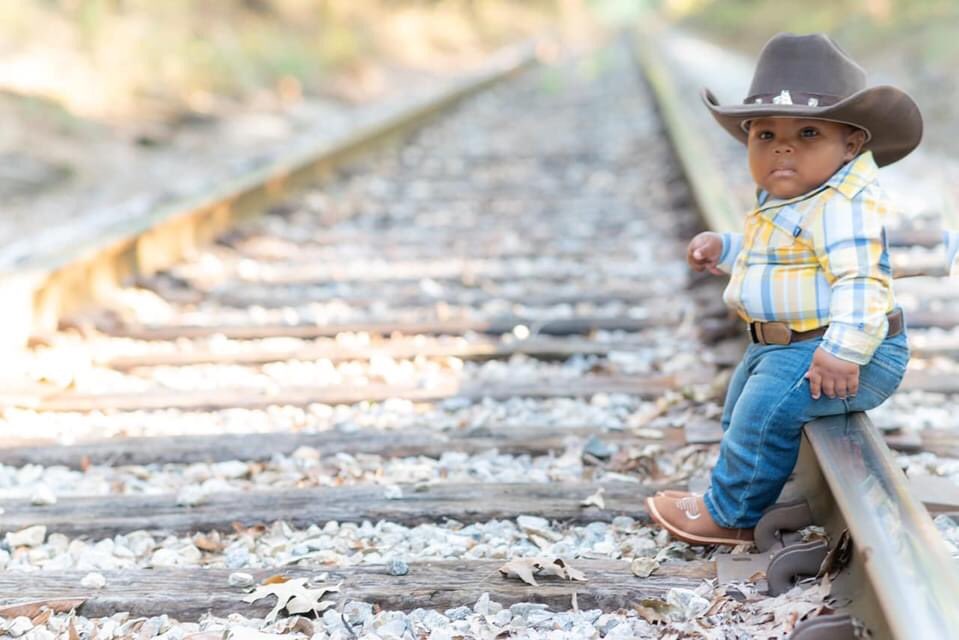In the image, a brown rope can be seen in the foreground, adding texture to the scene. The background is deliberately out of focus, emphasizing depth and drawing attention to the central subject. On the right side of the image, a very small child is seated on a metallic railway railing. The child is dressed in a charming ensemble: a black cowboy hat with a decorative band around its base, a black shirt adorned with multiple colors—white, blue, and yellow—a prominent belt buckle, blue denim jeans, and brown shoes. The railroad stretches from left to right, featuring metal railings and wooden boards that form the tracks, with gravel filling the spaces in between. The child, appearing slightly confused, gazes directly at the camera, adding an emotional touch to the photograph.